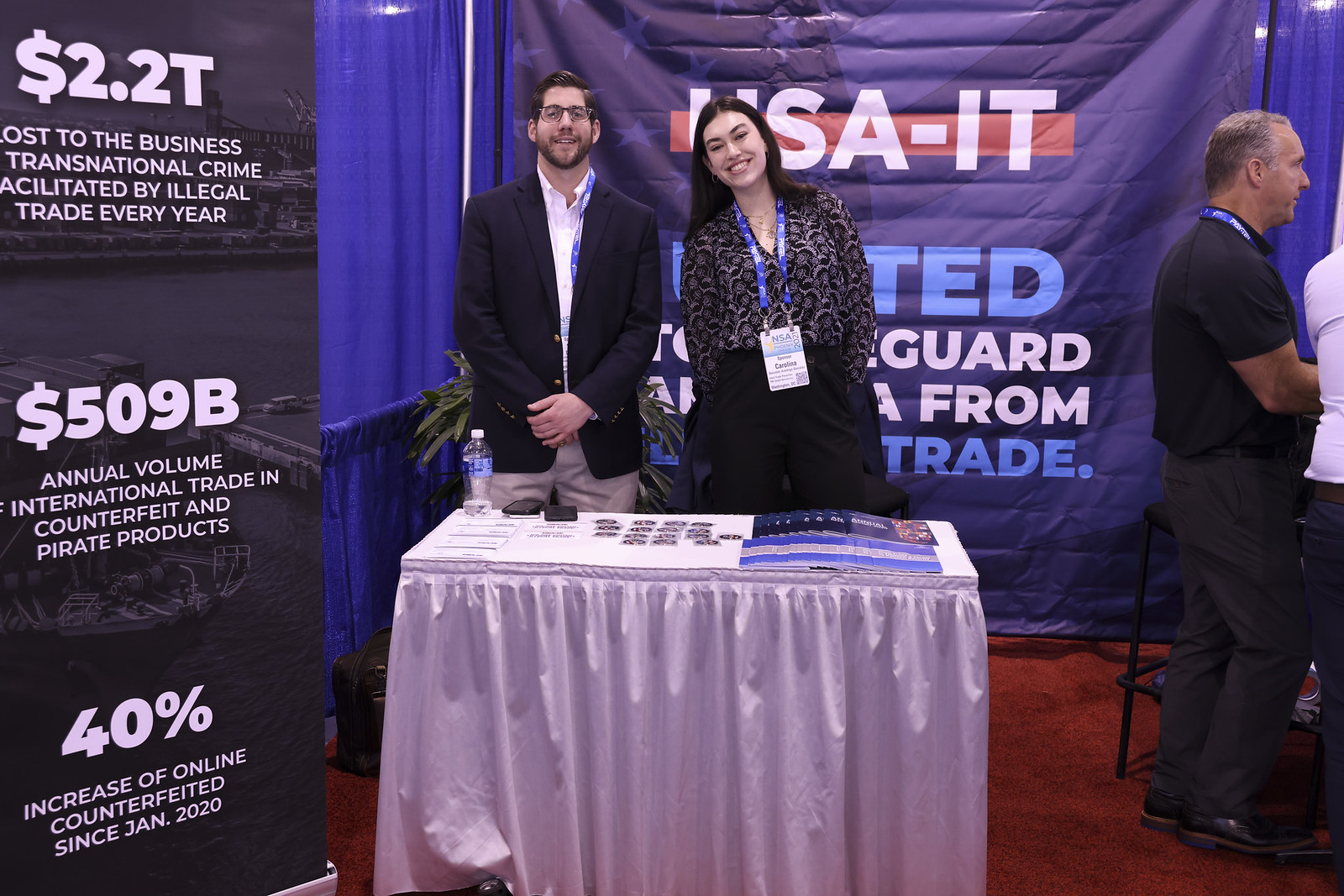This image showcases a booth at a trade fair or conference, with two people—one male and one female—standing behind a table adorned with a white tablecloth topped with a flowy skirt that touches the floor. The table displays blue brochures, white business or information cards, various stickers, and a water bottle on the left side. The man, who has fair skin, brown hair, glasses, a beard, and is dressed in a navy blazer, white button-down shirt, and khakis, stands to the left. The woman, with long dark hair, fair skin, and wearing a patterned black and white blouse, dark pants or a skirt, and a lanyard with a name tag, stands to the right, smiling with her head tilted towards her right. Behind them is a large blue banner with white and blue text accented in red. To the left, another banner with a dark photographic background and white text provides alarming statistics about illegal trade's impact on businesses: "$2.2 trillion lost to businesses transnational crime facilitated by illegal trade every year," "$509 billion annual volume of international trade in counterfeit and pirate products," and "40% increase of online counterfeiting since January 2020." These statistics are set against what appears to be an image of a barge departing a dock. Additional people are visible in the background, including a man in dark attire, all standing on a red shaggy carpet.